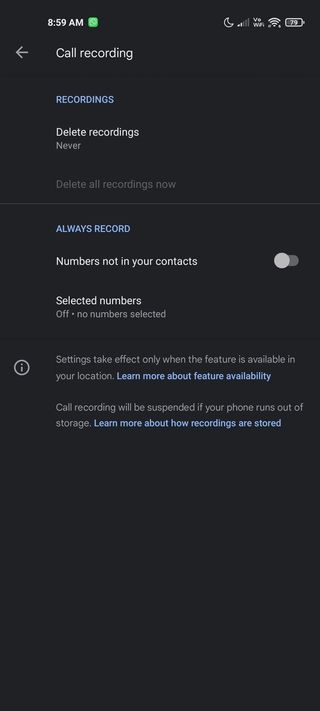The image is a screenshot taken from a smartphone showcasing the recording settings page, set against a completely dark background. 

At the top of the screen is the basic information bar typical of smartphones. On the left side, it displays the time as 8:59 AM, accompanied by a small green square. On the right side, there are five different icons, including indicators for wireless connectivity showing two out of five bars, and a battery icon depicting a 79% charge.

The main content of the page begins below this bar with the header "Call Recording" at the very top, which is preceded by a backwards arrow. Underneath the header, in light blue text, is the word "Recordings," indicating it is currently selected. Following this is the option "Delete Recordings" in white text, and directly below it, the word "Never" in gray, denoting its current status. 

A small space is followed by another grayed-out option "Delete All Recordings Now." A horizontal line spans the width of the screen to demarcate the next section. This section starts with the option "Always Record" in blue text. Just beneath this, the option "Numbers Not in Your Contacts" is visible in white text, paired with a toggle bar that is currently not selected. Below this, the option "Selected Numbers" is shown in white text, followed by the grayed-out text "Off" and "No numbers selected."

A dark line runs horizontally, segregating the bottom section of the page. This section begins with a disclaimer in two segments. The first segment states, "Settings take effect only when the feature is available in your location," accompanied by a circular 'i' icon for additional information. It also offers a clickable link to "Learn More about feature availability."

The second segment notes, "Call recording will be suspended if your phone runs out of storage," with an additional link in blue text that says, "Learn more about how recordings are stored," located directly beneath it.